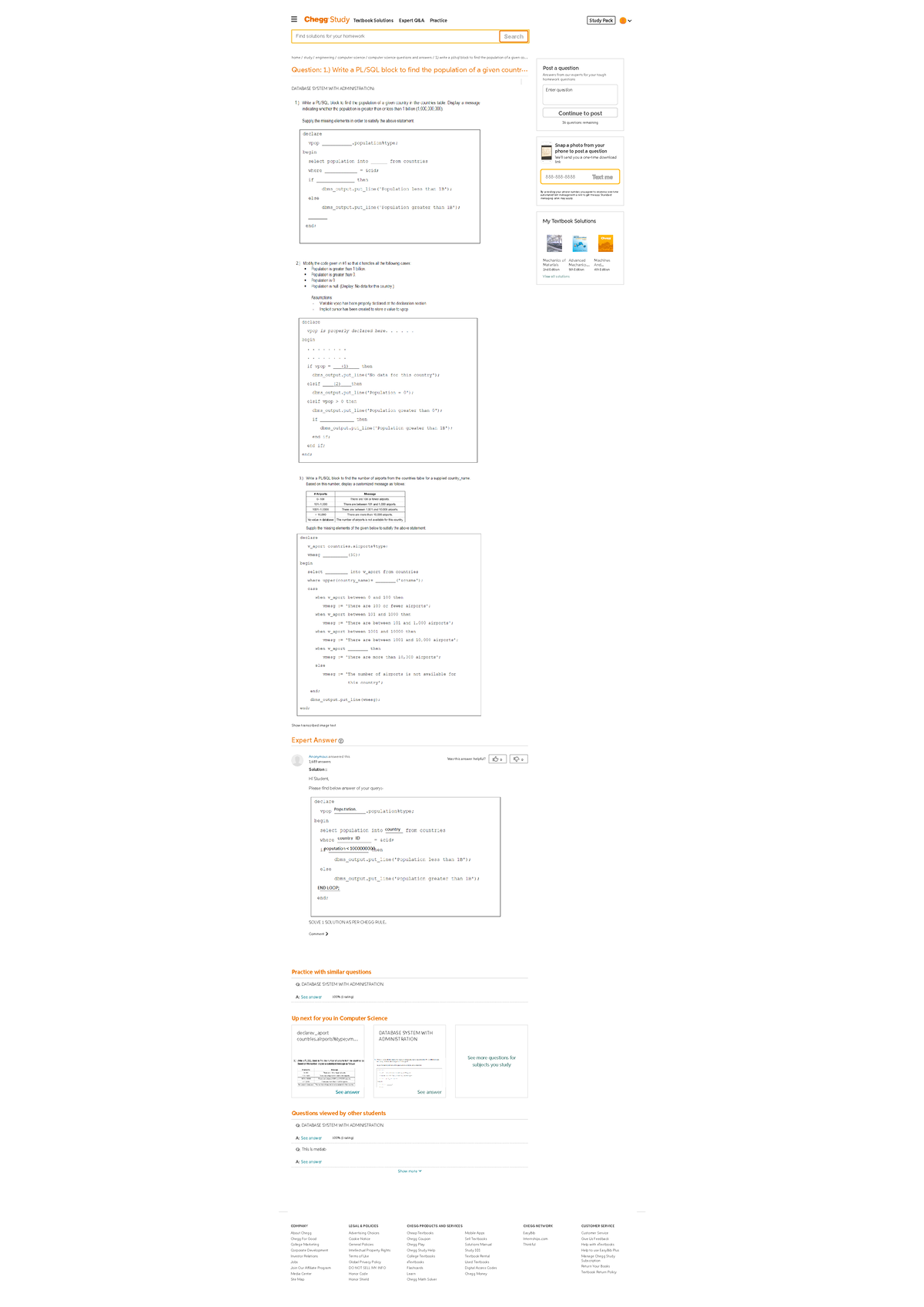In this image, we observe a webpage displaying academic content designed to assist students with their studies. Prominently featured is a search field at the top of the page, with the placeholder text "Find solutions for your homework." Just to the right of this search bar is a dropdown menu labeled "Study Pack." 

The main content area displays text sections with the following headings: "Check Study," "Textbook Solutions," and "Text Box Q&A Practice." Below this, we encounter the text for "Question One: Write a PL/SQL block to find the population of a given country." Beneath this question, there are several solutions provided, including an expert answer.

The color scheme of the webpage is highlighted by hues of orange, white, and blue, which are utilized to differentiate various sections and elements, enhancing readability and navigation.